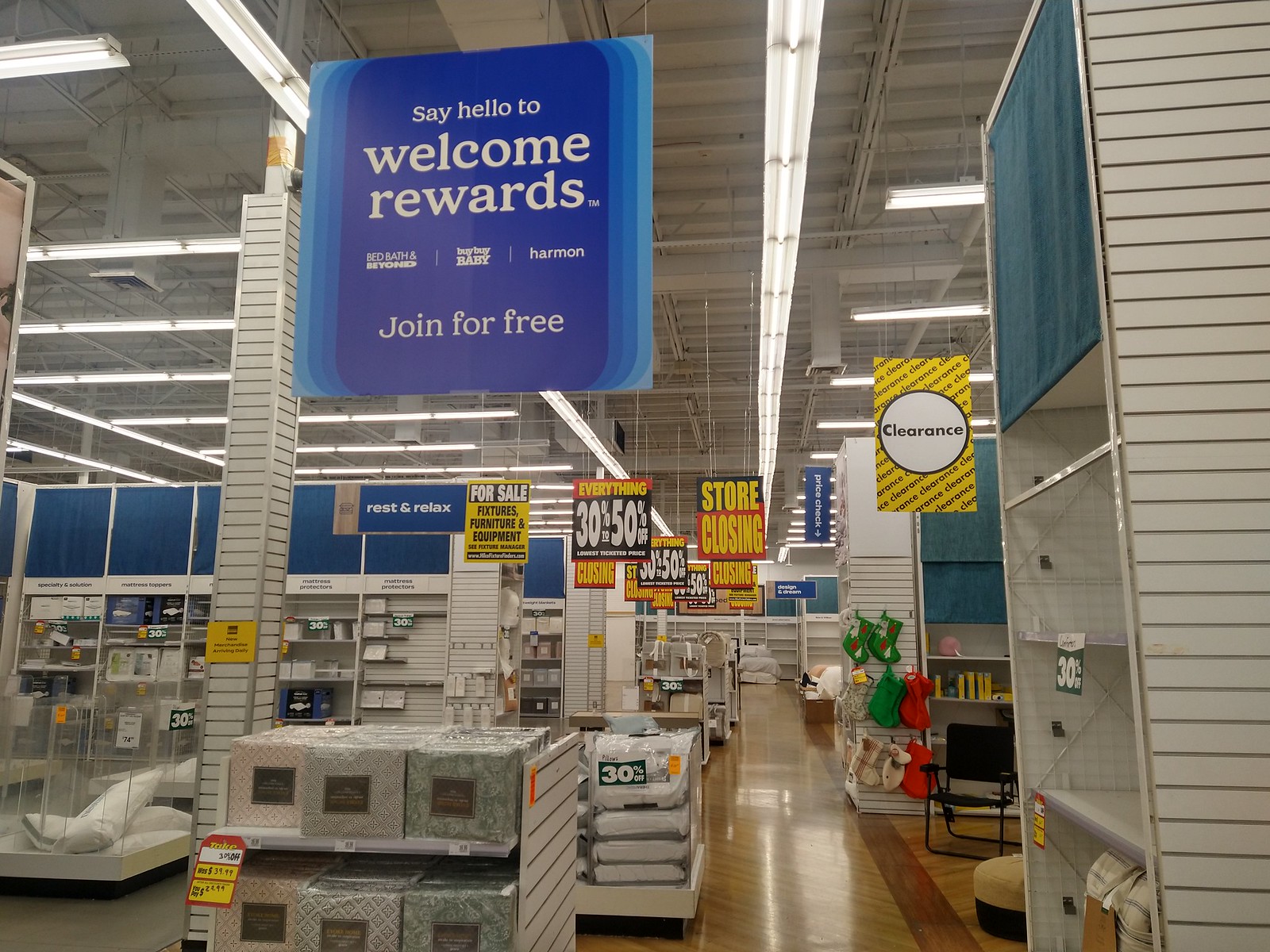The photograph, taken indoors, captures the bustling interior of a department store, likely a Bed Bath & Beyond. The store features light brown wooden flooring and a clean, minimalistic aesthetic with white walls and a white ceiling. Illumination is provided by large, white fluorescent lights that create a bright atmosphere. Hanging from the ceiling are several large, blue signs prominently displaying messages such as "Say Hello to Welcome Rewards," "Bed Bath & Beyond," "Harmon," and "Bed Bath Baby," with an invitation to "Join for Free" beneath.

Interspersed among these primary signs are a series of eye-catching yellow, black, and red signs boldly declaring "Store Closing," "Everything 30 to 50% Off," and "Clearance," indicating significant sales. The store is filled with numerous displays and shelves stocked with various household items, including pillows, sheets, and other home goods, providing a comprehensive shopping experience for customers. This detailed depiction highlights both the branding of the store and the current sales, drawing attention to its inviting and organized layout.